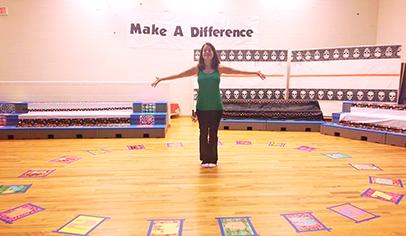This photograph features a Caucasian woman with brown shoulder-length hair standing barefoot on a hardwood floor, likely within a gymnasium or auditorium, distinguished by white walls and possible bleachers in the background. She is wearing a green sleeveless top and black yoga pants, standing with her legs together and her arms spread wide. Surrounding her on the floor are pieces of paper or drawings, each taped down in various colors—pink, yellow, green, and blue—forming a circle around her. Behind her, a banner with the words "Make a Difference" in black text is prominently displayed on the wall. Additional items, including steps and poster boards featuring repeated faces, are visible in the background. There is a bright light shining down, illuminating the scene, indicating it may have been taken casually and in an amateur style, possibly at a school or college campus involved in some philanthropical activity.